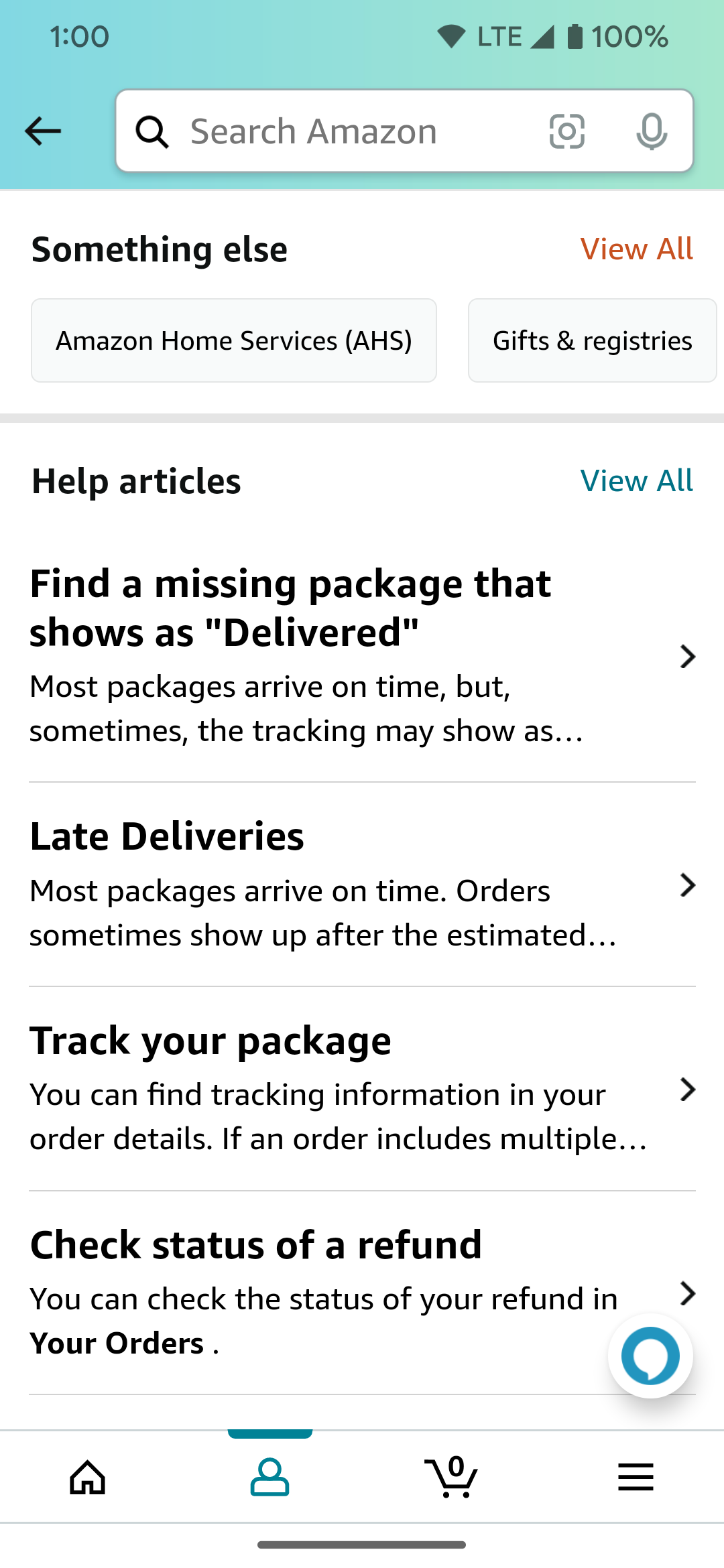This image displays a smartphone screen with a detailed interface. At the top, the screen indicates the current time as "1 o'clock" on the left, alongside symbols for full WiFi connectivity, LTE connection, full cellphone signal, and a battery level at 100%. Below that, there's a text field with the prompt "search Amazon."

The primary section of the screen pertains to Amazon Home Services (AHS), including categories such as "Gifts and Registries." There's a blue section labeled "Help Articles" with a specific mention of “Find Missing Packages.” A message displays stating "Most packages arrive on time, but sometimes check-in may show up," and it elaborates on occasional late deliveries, mentioning that "Orders sometimes show up after they're estimated."

Further information includes instructions to "Check-in package" and states, "You can find check-in information here," along with a note about checking package size and refi details. The bottom of the screen features several icons: a house icon on the far left, a blue person icon, a shopping cart icon, and a hamburger menu (three horizontal lines) indicating additional options.

A grey line separates the bottom icons from the rest of the screen, and a white bar is visible at the bottom, possibly indicating the virtual home button or navigation bar of the smartphone.